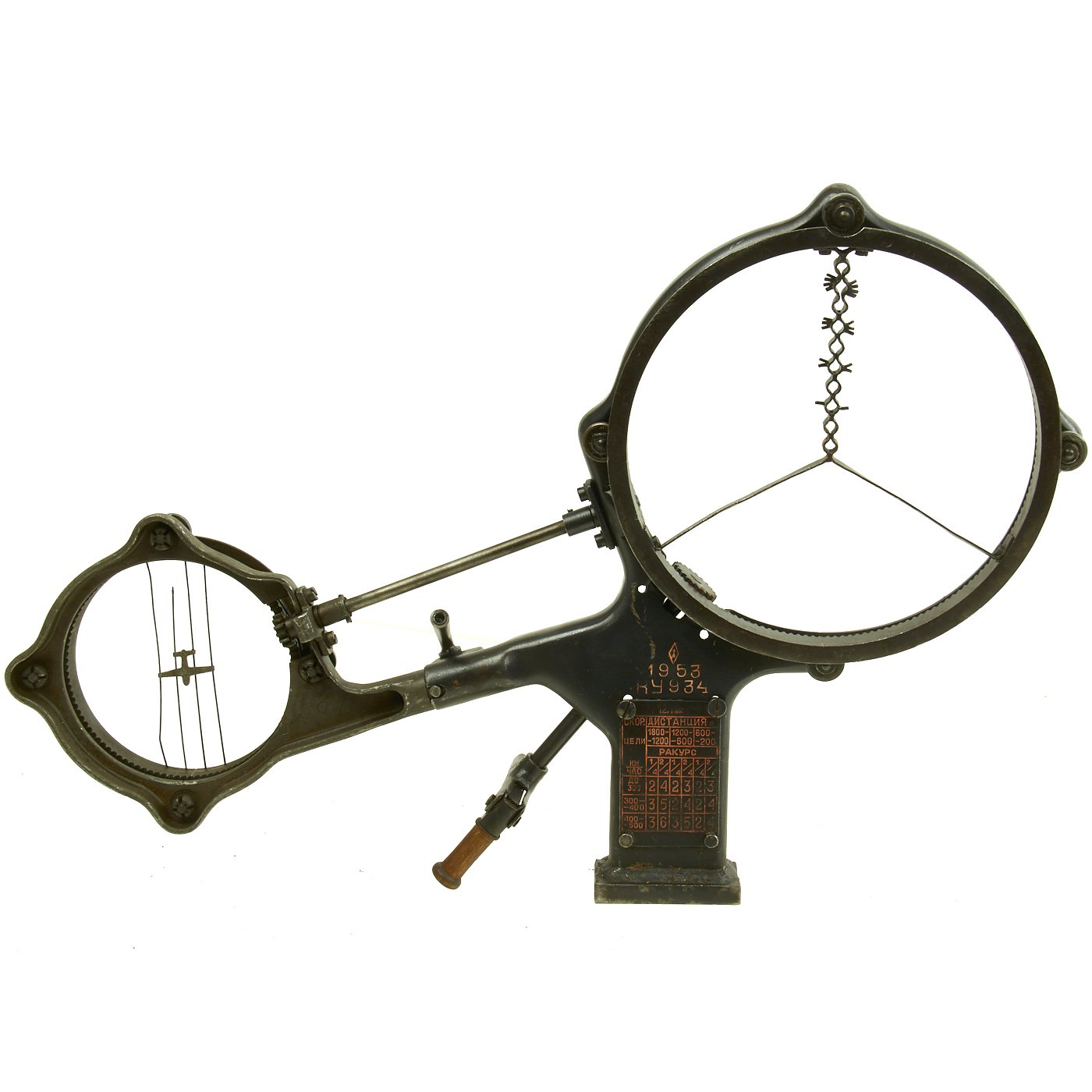The image depicts a detailed aviation instrument featuring two distinct circular components. The smaller circle on the left contains four vertical metal lines intersected by a silhouette of an airplane. The larger circle on the right displays a peace sign-like structure made from thin wire, with a center line that curls at the top, resembling barbed wire. Both circles are connected by two bars: a thick metal bar at the bottom and a thinner rod above it. The instrument rests on a black base, which supports these tilted circles. At the base, markings in a reddish color read "1953" along with additional numbers 1-9-5-3-4-8-3-4. There's also a hard-to-read graph below these numbers. A handlebar with a brown wooden grip extends from the left side of the instrument. The overall design suggests it could be an aviation device used to monitor distance or flight paths. Small notches are positioned at the north, east, south, and west points of each circle, adding to the instrument's intricate detailing.